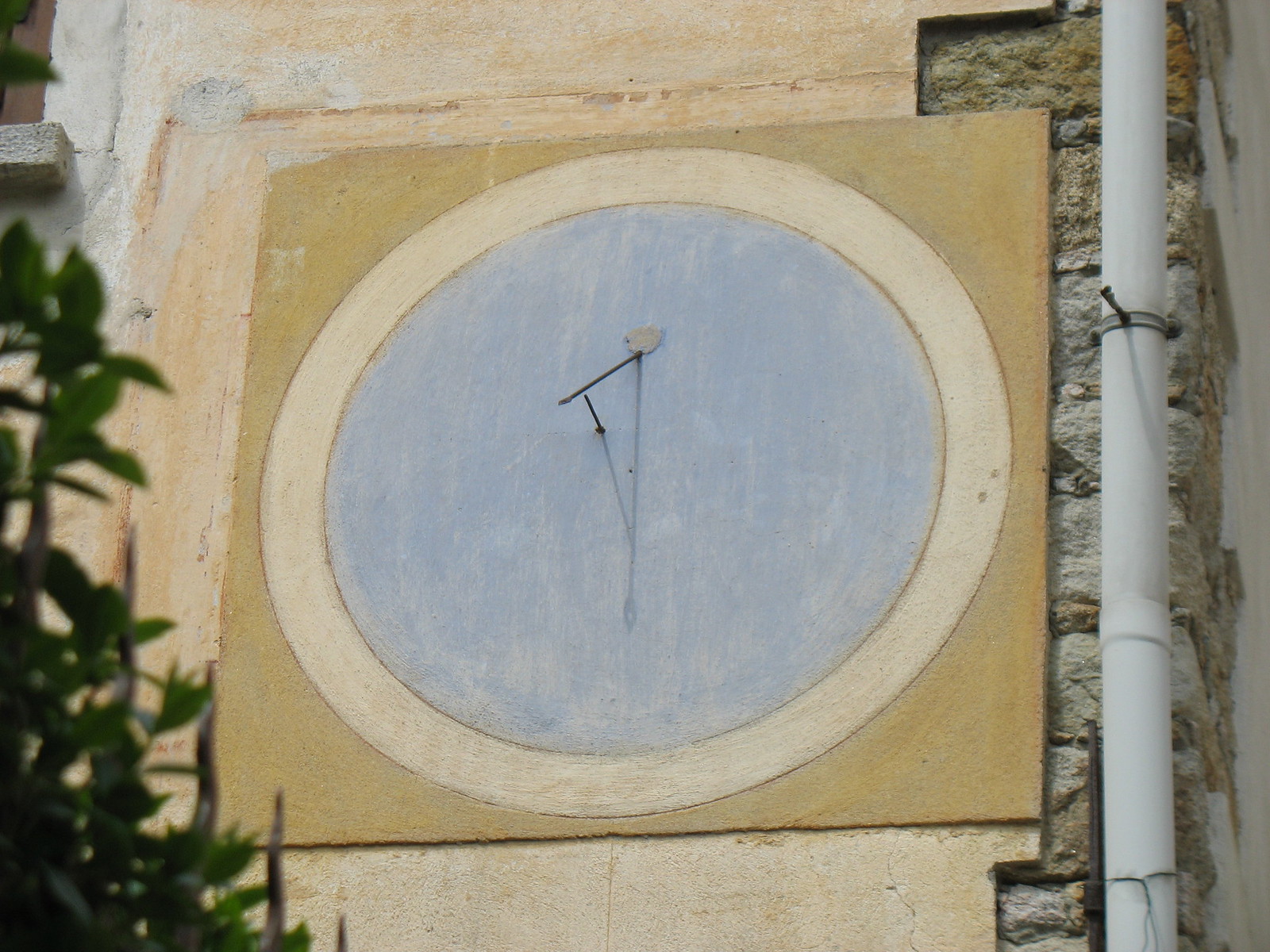The image shows an outdoor setting featuring a brick building with a lighter-colored brick background. Prominently displayed is a moderately sized, analog clock without any numbers or numerals. The clock has a blue face and is encircled by a beige border, which is further framed by a square brown border. The clock indicates the time as 8:30, judged by the positions of the hands—one of which appears intact while the other might be broken or missing. Mounted on the wall, the clock is affixed by a grip secured with bolts. Near the base of the clock is a metal projection, and a gray or white cylindrical pole adds structural support. In the image foreground, part of a tree or green bush is visible to the left, enhancing the outdoor atmosphere.